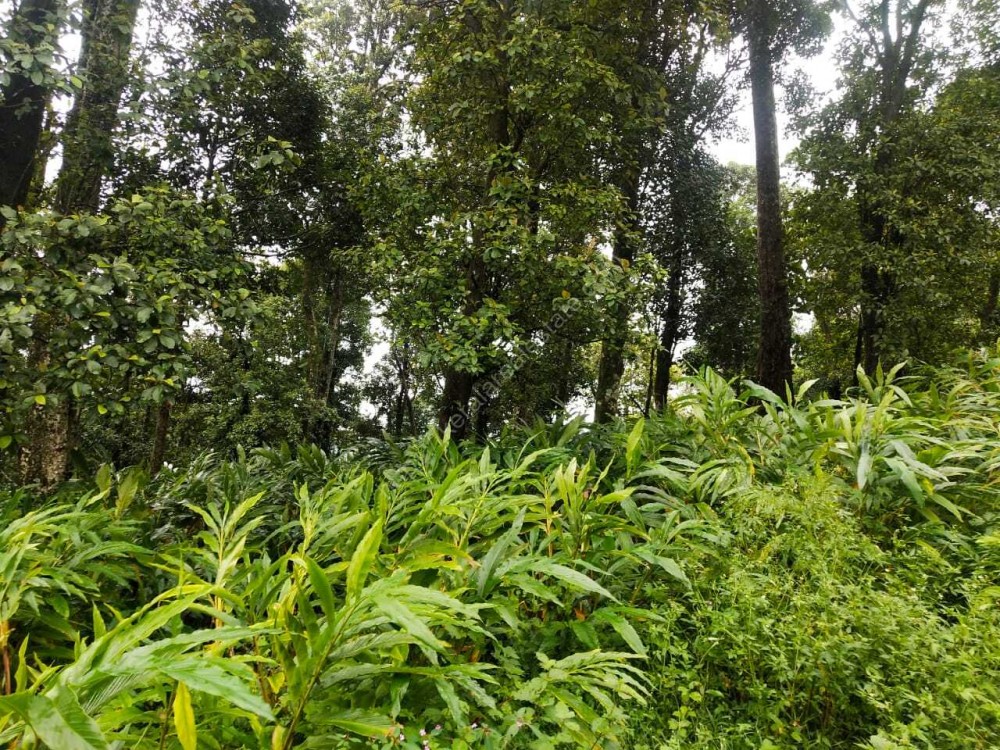The photograph captures a dense, lush green outdoor nature scene dominated by a variety of leafy plants and trees. In the background, a collection of very tall trees with bare trunks and sparse lower branches towers over the scene, suggesting a forest or jungle setting. The trunks are brown and extend high into the sky, which is visible through gaps in the foliage and appears white or gray, indicating an overcast day. In the foreground, there are shorter, unkempt leafy bushes of various heights, some with small and thin leaves. The overall impression is a vibrant wall of green hues, punctuated occasionally by hints of yellow, but devoid of any animals, flowers, or other noticeable objects.